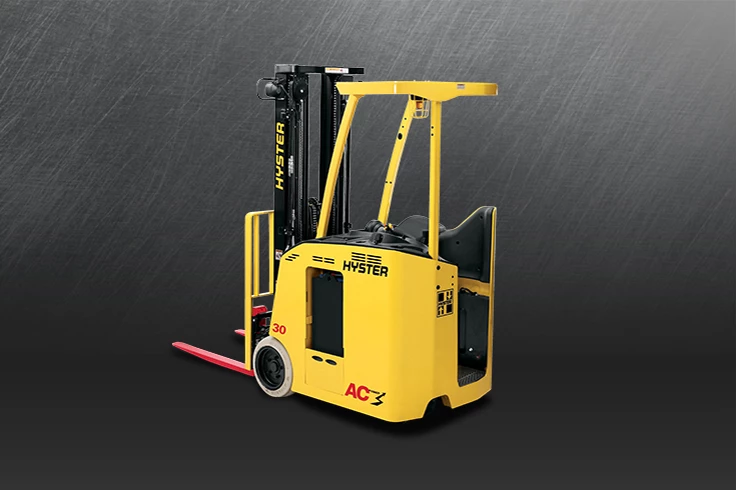This photograph showcases a bright yellow Hyster forklift against a black backdrop that has a slightly scratched, almost rain-like texture in some areas. The forklift, designed for standing operation, features a black hydraulic lift mechanism emblazoned with the Hyster logo in yellow, written vertically. The prongs for lifting are painted a vivid red, while the small wheels are gray with black rims. Prominently displayed near the front wheel is the number '30' in red. On the left side of the forklift, near the top, 'Hyster' is written in black text, while below this, 'AC' and a blue arrow symbol are visible. The forklift's support structure includes three yellow bars leading up to a flat surface and a caged red light within the cabin area. The specificity of details, such as the red '30' and the design elements, suggests the forklift is a newer model placed in a visually controlled setting for the photograph.